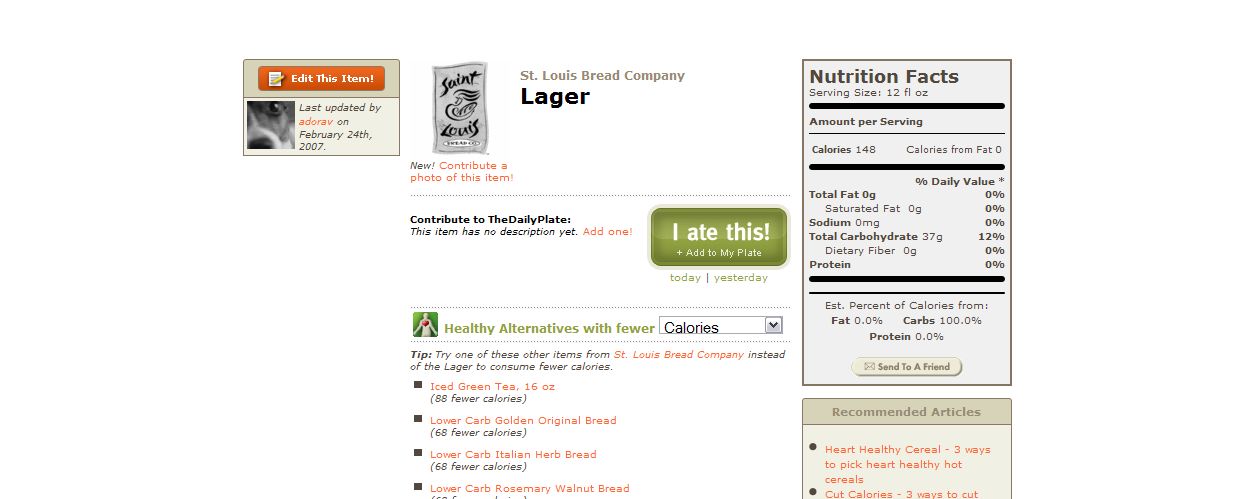This image is a screenshot from a diet or food nutrition app, last updated by Adorav on February 24, 2007. It prominently features a detailed view of a product from the St. Louis Bread Company—specifically, their Lager beer. On the left is an orange "Edit this item!" box, and below it, prompts for users to contribute information, including a photo upload option. In the center, there are detailed nutritional facts for the Lager: 148 calories per 12 fluid ounces, zero fat, with related information about carbs, sodium, and protein. A green button labeled "I ate this!" allows users to add the item to their food planner. The app also suggests healthier alternatives with fewer calories, such as iced green tea (88 fewer calories), and various lower-carb bread options. The interface includes a drop-down menu for filtering alternatives by different nutritional criteria like calories, fat, or salt content. Additional features include links labeled "Today" and "Yesterday" for easy tracking, and sections for user-contributed descriptions and tips.